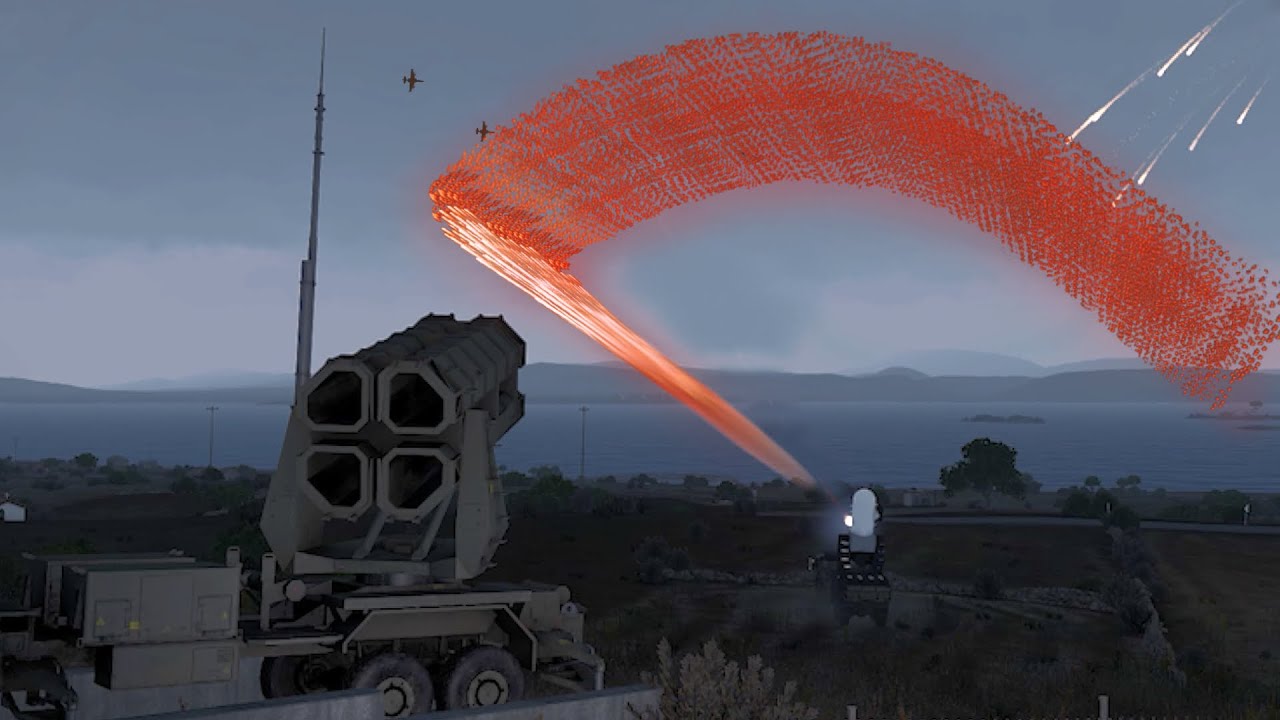The photograph depicts a dramatic coastal battlefield scene at either sunrise or sunset, characterized by its dark, dusky tones. In the foreground to the left, there is a prominent military vehicle equipped with large artillery machinery, aiming towards a serene bay that stretches to distant mountains. Adjacent to the vehicle, an ambiguous, large, pointy object is visible. The sky features two fighter jets and an arc of bright red light, possibly from gunfire or missiles, captured in a striking time-lapse effect. In the upper right corner, there appears to be multiple streaks of light resembling shooting stars or perhaps a burst of fireworks, adding an unexpected visual element. The image combines eerie calmness with intense military activity, creating a puzzling yet captivating composition.